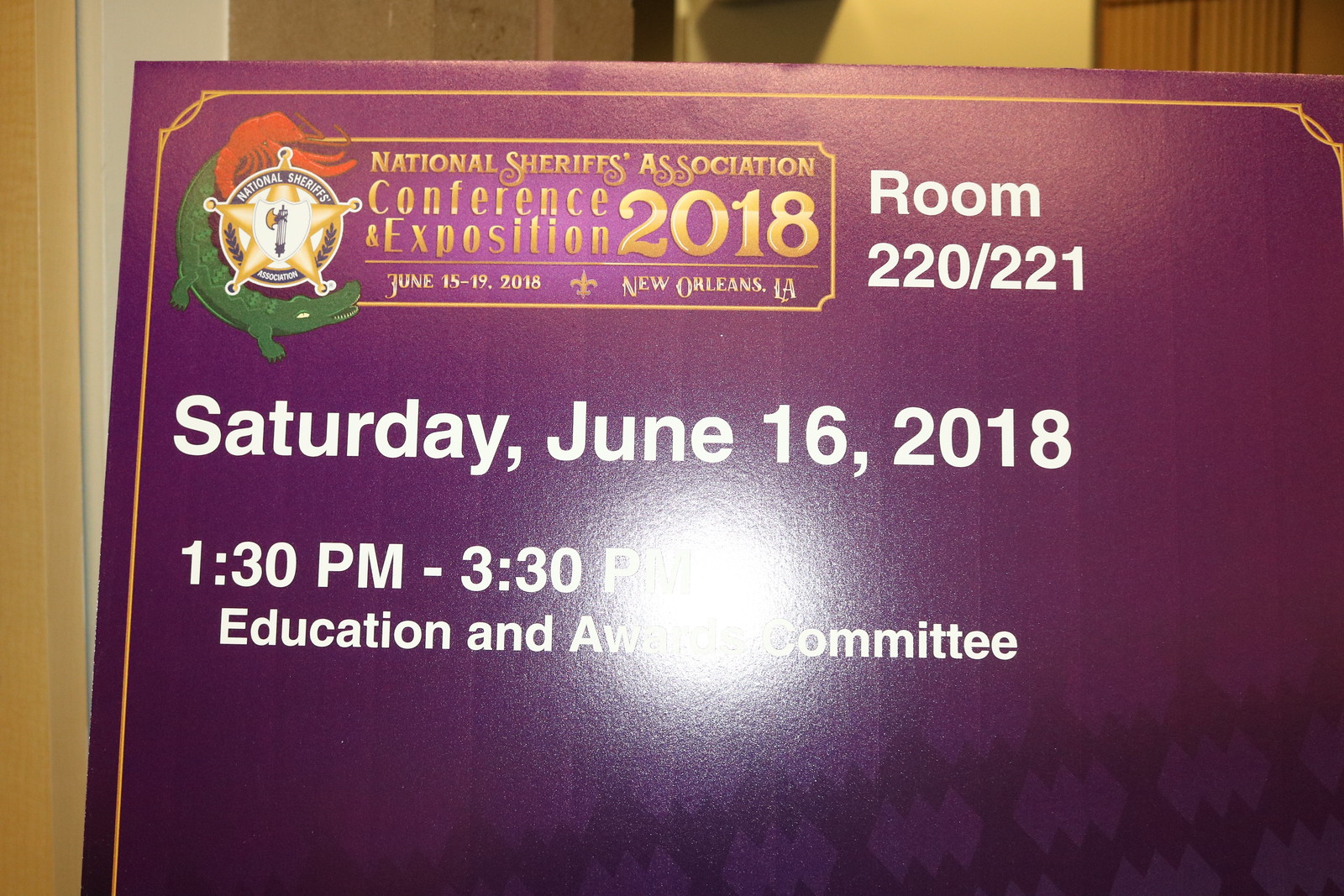The image depicts a thick, rectangular, dark purple sign or billboard with gold edges. Prominently displayed in the upper left corner is the emblem of the National Sheriff's Association, featuring a gold sheriff's badge entwined with a green alligator. The sign reads: "National Sheriff's Association Conference and Exposition 2018, June 15-19, 2018, New Orleans, Louisiana." To the right of the logo, it specifies the location "Room 220-221" and the event details: "Saturday, June 16, 2018, 1:30 p.m. - 3:30 p.m., Educational and Award Committee." The image contains a noticeable white camera glare in the center.